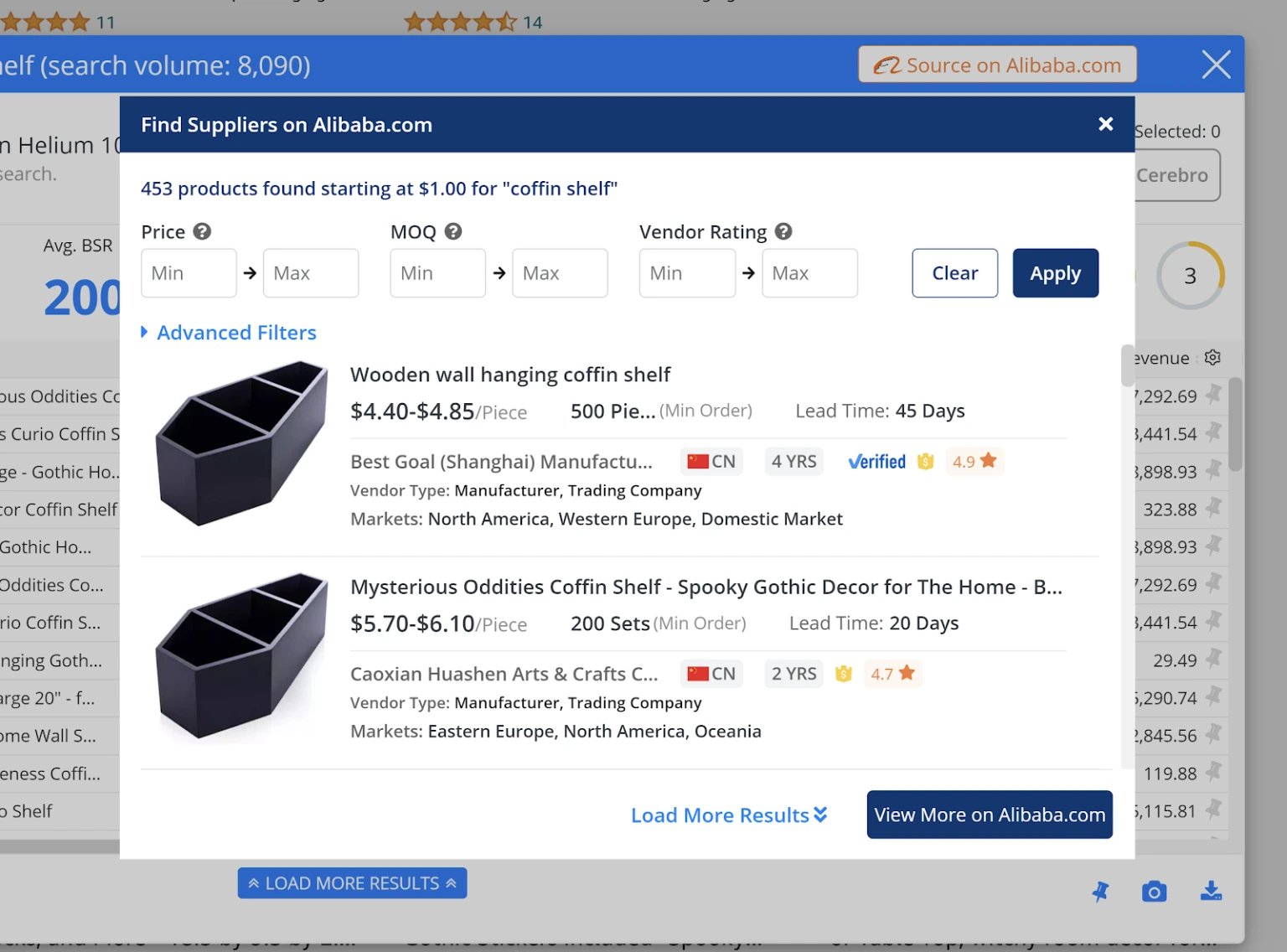This image shows a detailed product listing on Alibaba.com for decorative wooden coffin shelves. The focal point of the screen displays a black wooden coffin shelf, highlighted with text describing its price range of $4.40 to $4.85 per piece, with a minimum order requirement of 500 pieces. The listing indicates a lead time of 45 days, and the supplier, Best Gold Shanghai Manufacturing, is verified and has been operating for four years.

In the background, a secondary product listing for a Mysterious Oddities Coffin Shelf is visible, labeled as spooky gothic decor for the home. This alternative product is priced between $5.76 and $6.10, with a minimum order quantity of 200 pieces and a lead time of 20 days.

The interface includes options to load more results or view additional details on Alibaba.com, with filters like minimum and maximum price, vendor rating, and advanced filtering tools clearly displayed. The user is prompted to clear and apply these search parameters. The overall effect of the image is somewhat eerie due to the nature of the product, which serves as a decorative piece for those interested in gothic and mysterious home decor.